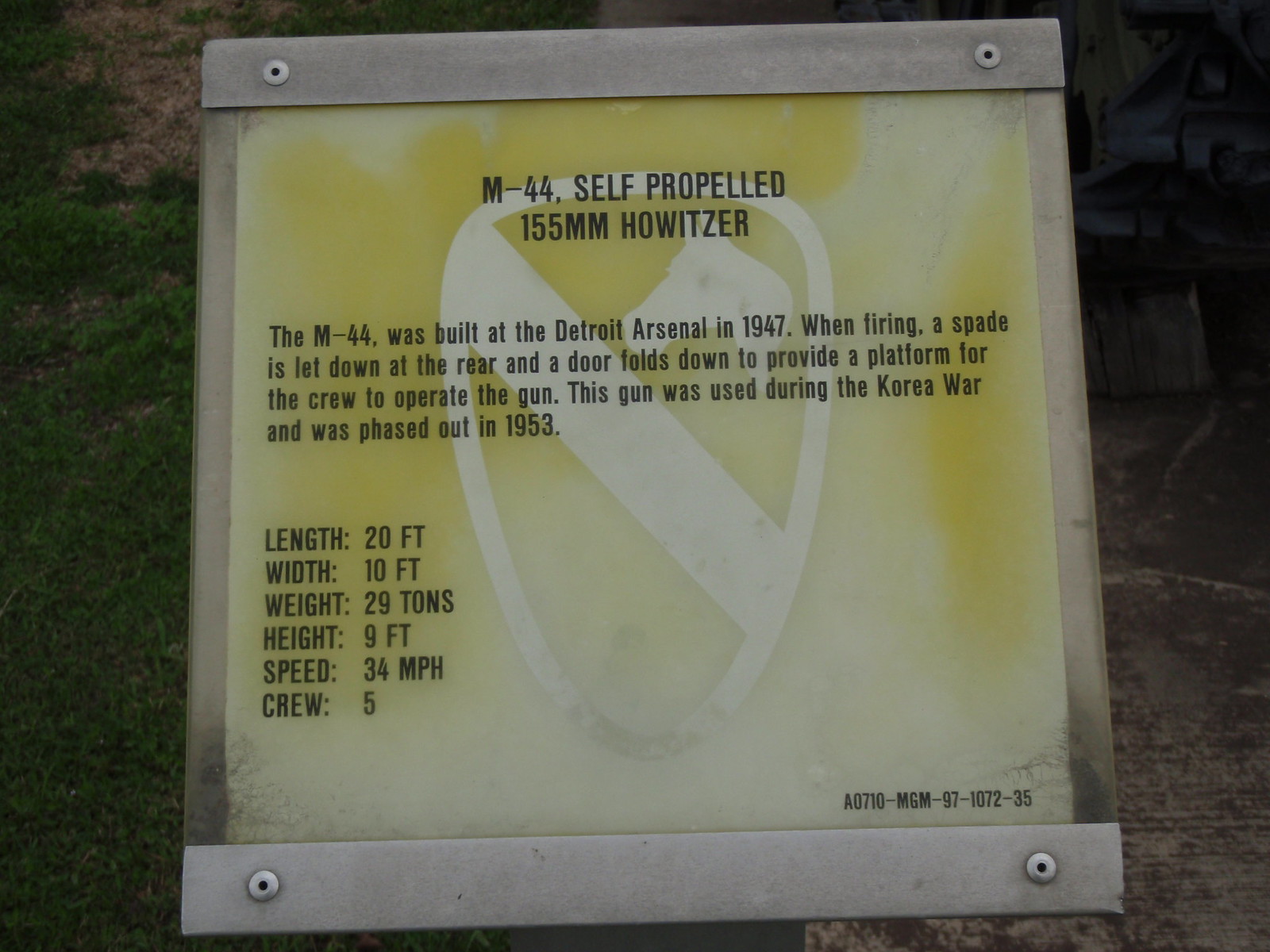This image features an outdoor plaque set against a backdrop of greenery and stone. The plaque is made of glass with a faded yellow tint and is framed with metal rivets at the top and bottom, securing it in place. Prominently displayed in the center of the plaque is a shield-like logo depicting a horse’s head facing left, set within an oval shape, with a banner diagonally across it.

The plaque bears the title "M-44 Self-Propelled 155mm Howitzer" in bold black lettering. Below the title, an informative block of text explains that the M-44 was built at the Detroit Arsenal in 1947. It details that during firing, a spade is deployed at the rear, and a door folds down to provide a platform for the crew to operate the gun. The M-44 played a significant role during the Korean War and was phased out in 1953.

On the left side of the plaque, key specifications of the M-44 are listed: 
- Length: 20 feet
- Width: 10 feet
- Weight: 29 tons
- Height: 9 feet
- Speed: 34 mph
- Crew: 5

In the bottom right corner, an item number is displayed: A0710-MGM-97-1072-35. The background visible in the image shows a darkened outdoor environment with grass and dirt, emphasizing the outdoor setting of this exhibit.